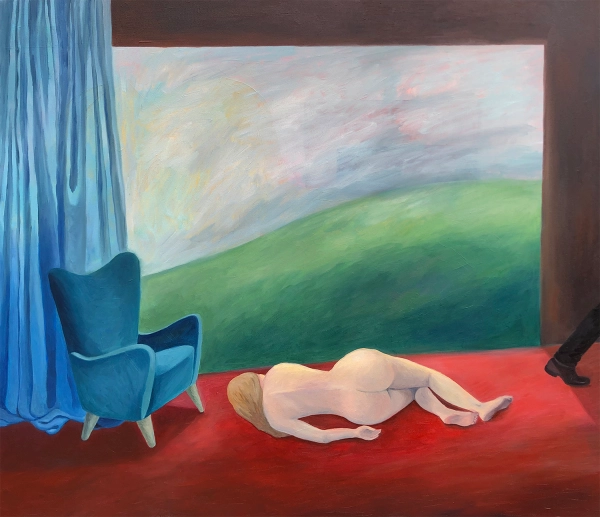The painting depicts a nude woman lying on a red carpeted floor with her back towards the viewer. Her long blonde hair is tucked under her shoulder, and her left arm is wrapped behind her, accentuating her shapely figure and bare buttocks. Her legs are slightly bent, and the bottoms of her feet are visible. She is positioned in the lower middle portion of the painting, close to a blue chair with wooden legs near her head. A blue curtain hangs from the left side of the painting, extending from the floor to the top of the painting.

Surrounding the scene is a brown wall featuring a picture window or open space that reveals a daytime landscape with green grass and a hill under a sky with hues of orange and blue, suggesting it might be late afternoon. To the right of the woman, a black-clad leg and foot, appearing to walk away, are partially visible, exiting the right edge of the painting. The painting lacks a signature and date.